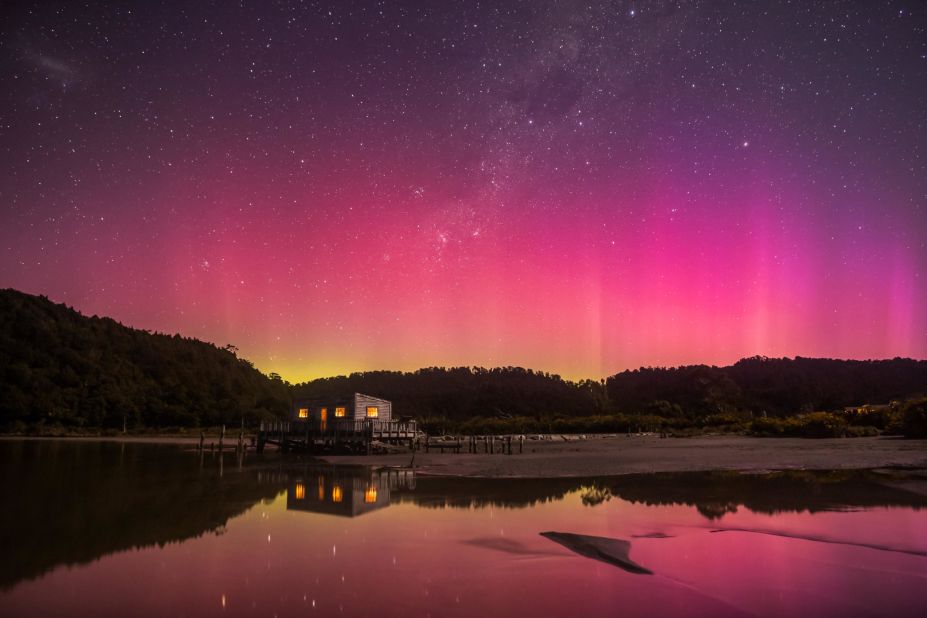This captivating color photograph portrays a small, remote cabin built on stilts over a tranquil lake, surrounded by a dense tree line with no other houses in sight. The scene is bathed in the vivid hues of a post-sunset sky, with shades of pink, orange, purple, and a hint of yellow creating an almost surreal backdrop. Every light inside the cabin is turned on, casting a cozy glow that contrasts beautifully with the night sky. The lake's mirror-like surface reflects the majestic sky and the illuminated cabin, enhancing the surreal, almost airbrushed quality of the image. The stars are faintly visible in the colorful sky, adding a touch of serenity to the picturesque setting. A silhouette of trees forms a dark outline against the radiant sky, completing this very detailed and vivid portrayal of a serene lakeside evening.